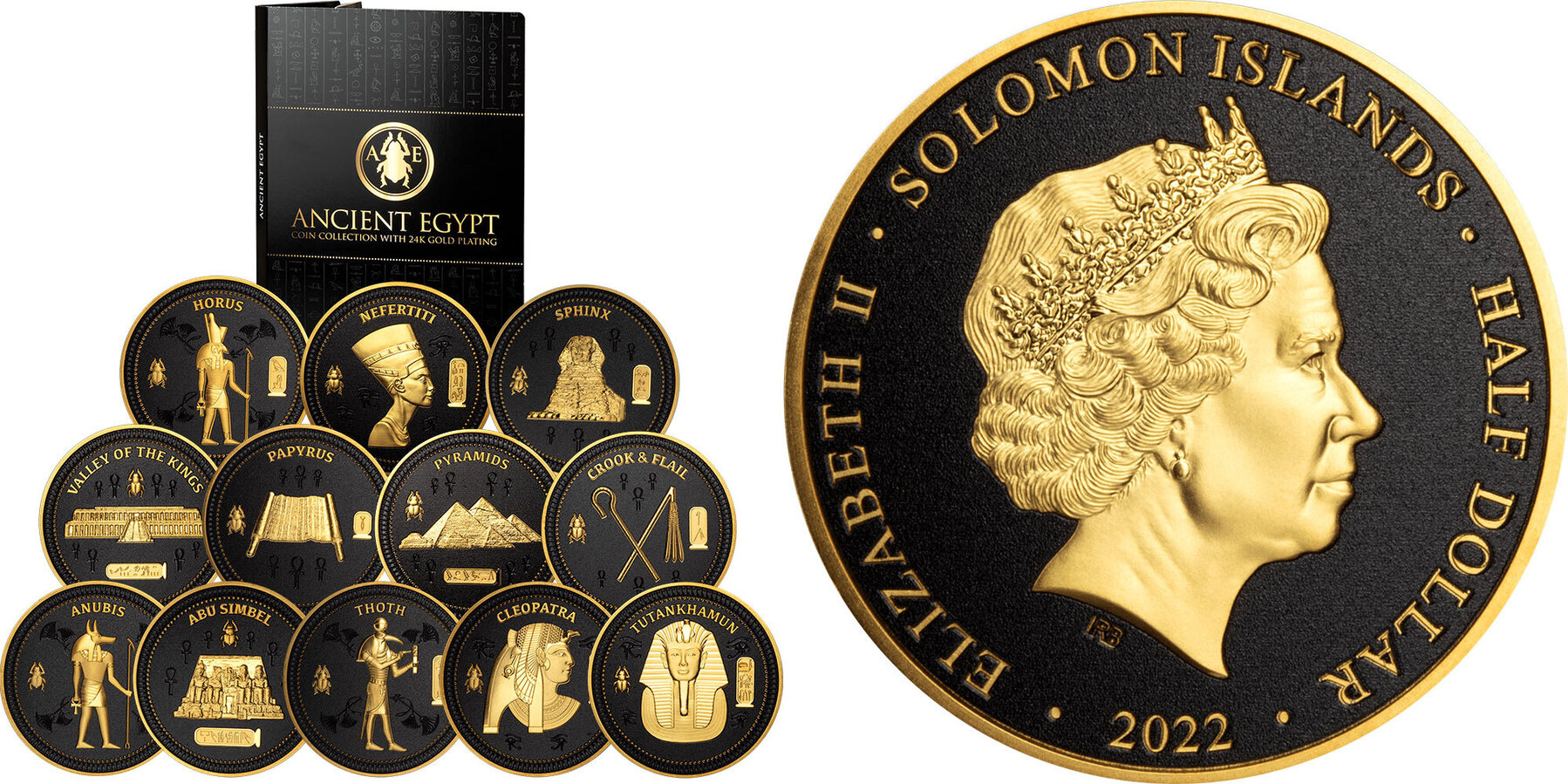The image showcases a detailed coin collection featuring 13 coins, with a prominent focus on a commemorative coin from Solomon Islands celebrating Queen Elizabeth II. This main coin is striking with its black background, gold border, and a gold portrait of the Queen looking to the right. Inscribed in gold around the coin are the words "Solomon Islands, Elizabeth II, Half Dollar, 2022." Next to this coin, towards the left, lies a sleek black case titled "Ancient Egypt" in gold, adorned with a gold beetle and the letters "AE".

Below the case, twelve additional commemorative coins are neatly arranged in three rows—three coins on the top row, four in the middle, and five at the bottom. Each of these coins mirrors the main coin in design, featuring a black background with a gold border and gold illustrations that depict various iconic Egyptian symbols and figures. The coins are labeled with terms such as "Horus," "Nefertiti," "Sphinx," "Valley of the Kings," "Papyrus," "Pyramids," "Crook and Flail," "Anubis," "Abusimbel," "Thoth," "Cleopatra," and "Tutankhamun," each accompanied by corresponding golden images. The cohesive gold and black color scheme exudes a rich, historical elegance, anchoring the collection in its ancient Egyptian theme.